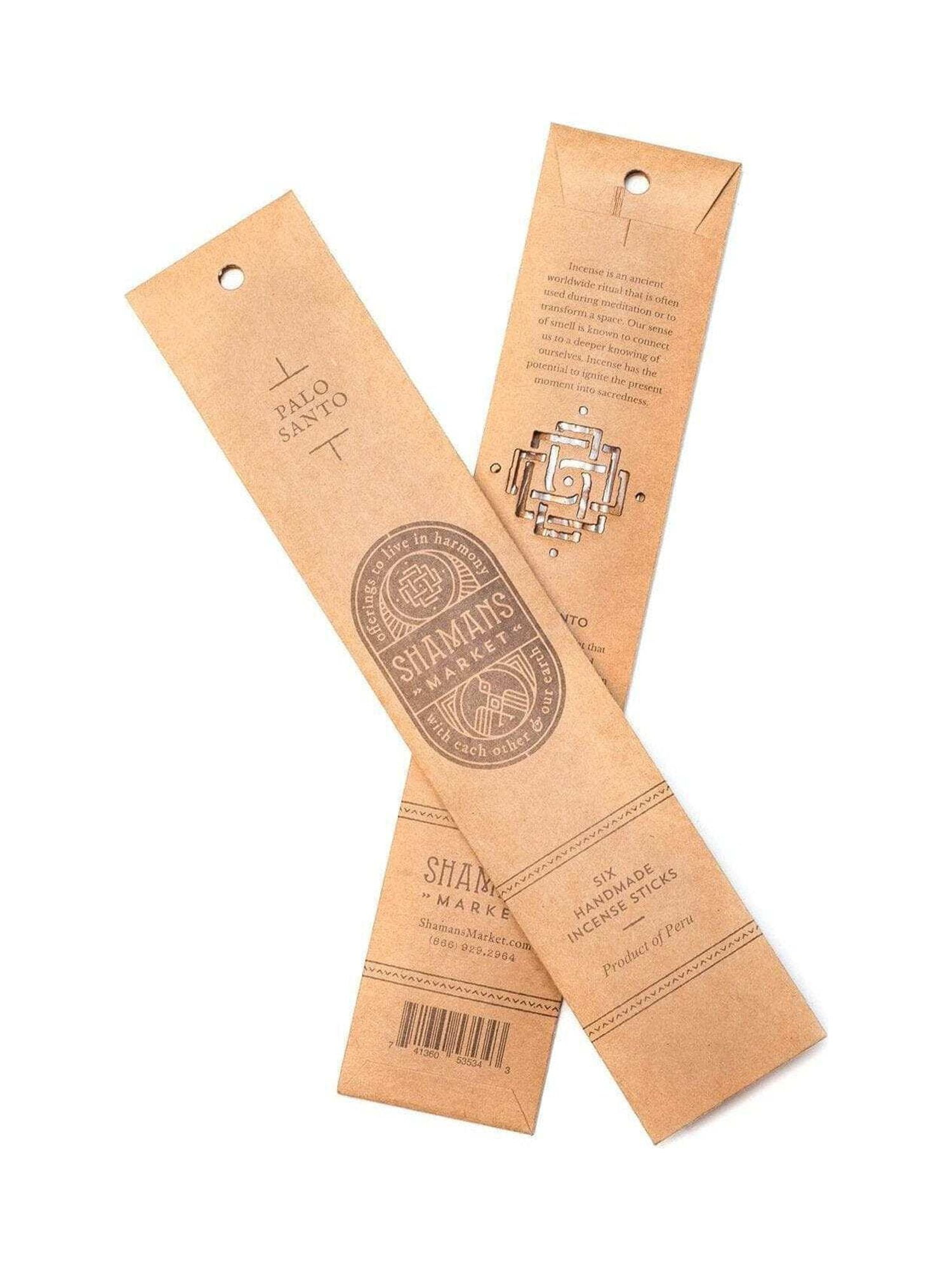The image depicts two cardboard packages of incense sticks positioned one over the other, arranged diagonally from the top left to the bottom right. The packaging is slim, rectangular, and beige with brown text and intricate Native American designs. The top package features the scent "Palo Santo" along with the brand name "Shaman's Market," accentuated with symbolic arrows around the name. Additionally, it states, "Offering to Live in Harmony With Each Other and Our Earth." The bottom of the package reads, "Six handmade incense sticks, Product of Peru," and includes a tribal bird logo.

The text on the front also mentions the ritualistic nature of incense, emphasizing its historical usage in meditation and space transformation. This underscores the connection between the sense of smell and a deeper understanding, highlighting its potential to infuse sacredness into the present moment.

The back of the package reveals a partially visible barcode, the repeated brand name "Shaman's Market," the website "shamansmarket.com," and some additional text obscured by the overlap. The overall presentation suggests these incense sticks are not only functional for meditation but are also crafted with cultural significance in mind, offering a glimpse into Peruvian craft and spirituality.